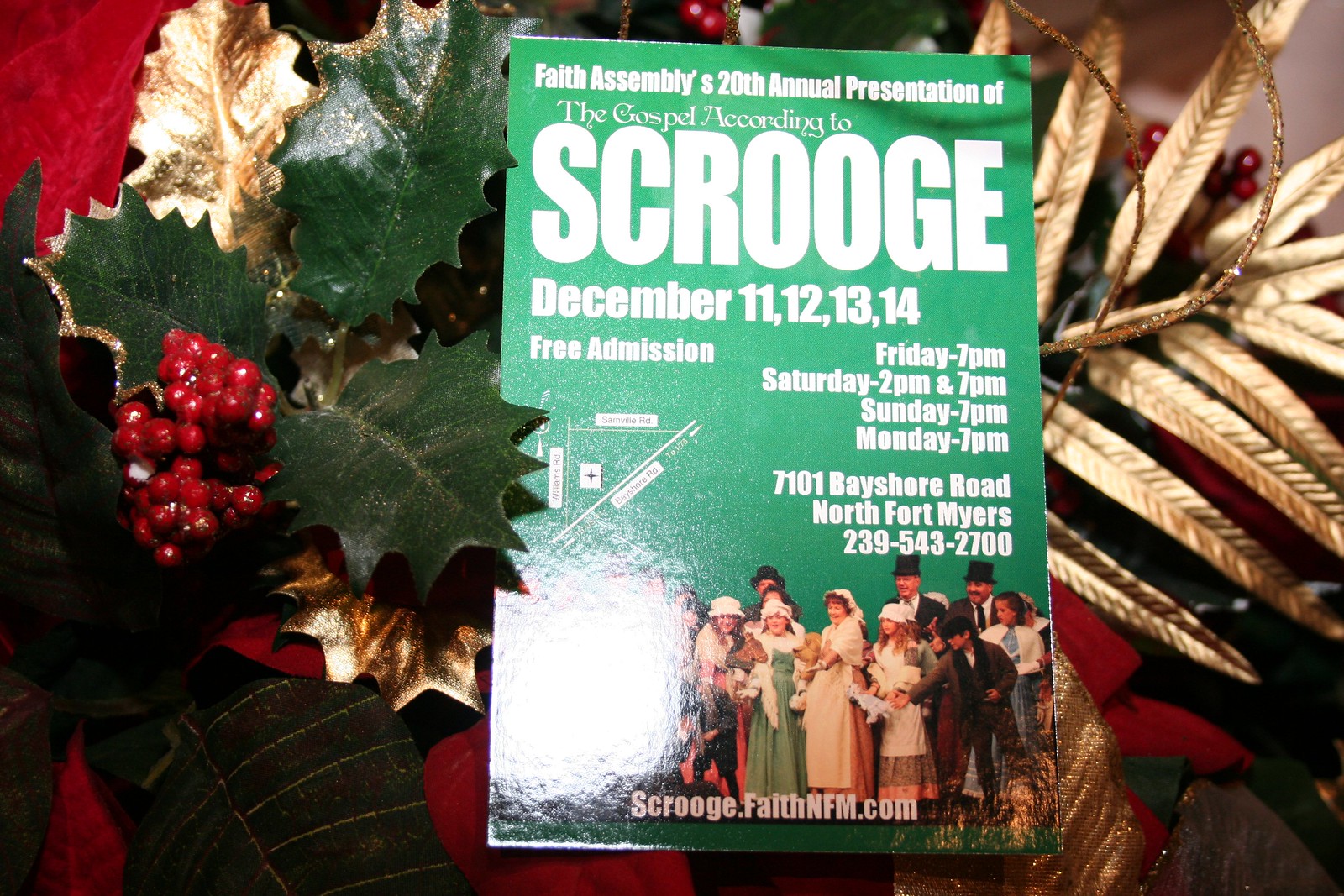The image portrays a festive Christmas scene featuring a decorative arrangement with mistletoe, holly, red berries, and gold leaves, accentuating a prominently displayed green poster. At the top of the poster, in bold white text, it announces, "Faith Assembly's 20th Annual Presentation of the Gospel According to Scrooge," with "Scrooge" emphasized in large, capitalized letters. The event dates, "December 11, 12, 13, 14," are listed below, followed by "free admission." The schedule indicates showtimes: Friday 7 p.m., Saturday 2 p.m. and 7 p.m., Sunday 7 p.m., and Monday 7 p.m. Further down, the location and contact details are provided as "7101 Bayshore Road, North Fort Myers, 239-543-2700." Additionally, a web address, "Scrooge.FaithNFM.com," is noted. At the bottom of the poster, a group of actors in period costumes are posing, with women in white headscarves and long dresses, and men in tall black hats, suits, and ties. A significant glare affects the left side of the poster, partially obscuring some information.